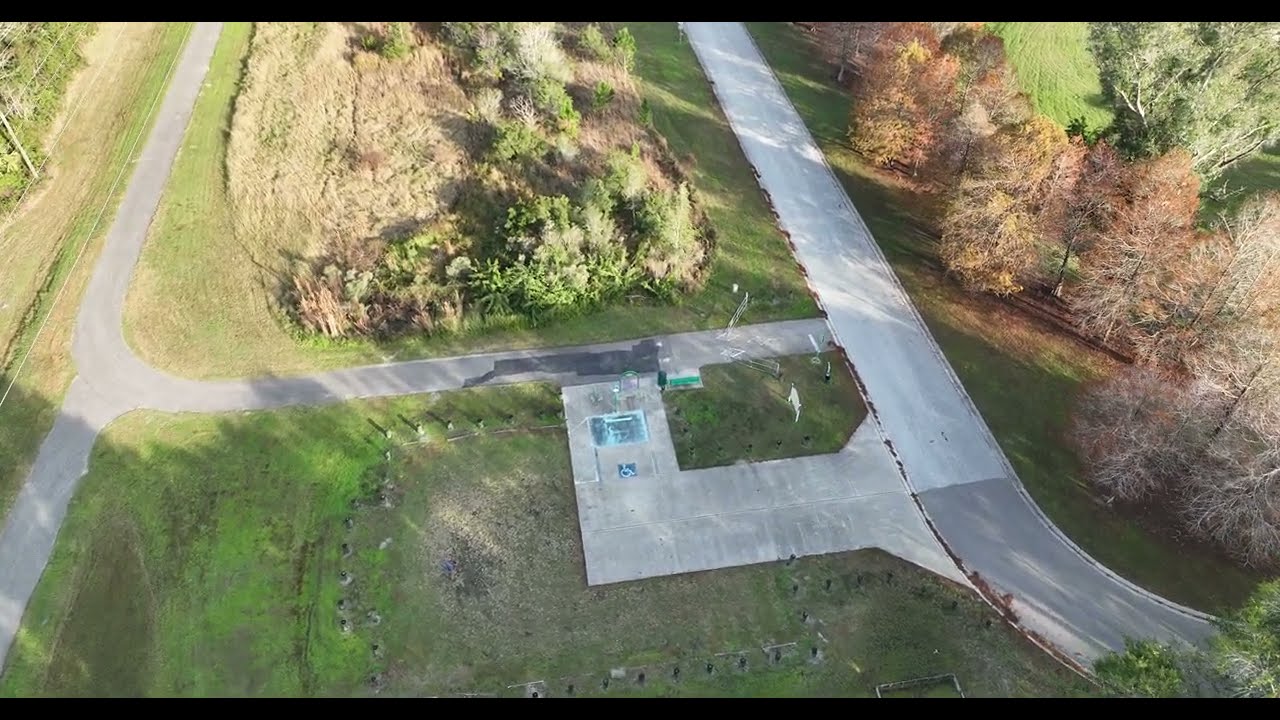This overhead aerial shot, captured by a drone during the daytime, presents a sprawling grassy region with a network of winding, gray roadways forming an H-like pattern. This intricate roadway comprises a left stretch running from top to bottom, a middle stretch bisecting the image, and a right stretch also extending top to bottom before curving out to the right. The scene is rich in greenery, featuring numerous tall trees with varied hues - vivid green trees, red trees, some brown, and others grayish-white. Among these trees, there are patches of grass, some green and lush, while others appear patchy, worn out, and intermixed with dirt and debris, suggesting seasonal changes like winter. 

In the center of this area, an L-shaped gray pavement is noticeable, containing a blue object that resembles a swimming pool. Adjacent to this pavement on the foreground, remnants indicate a previously existing structure, possibly a house, now indicated by posts and a stretch of concrete leading to a handicapped parking space symbol. The absence of lane delineations on these narrow yet winding streets adds a sense of confusion on how traffic navigates this tranquil yet somewhat desolate landscape.